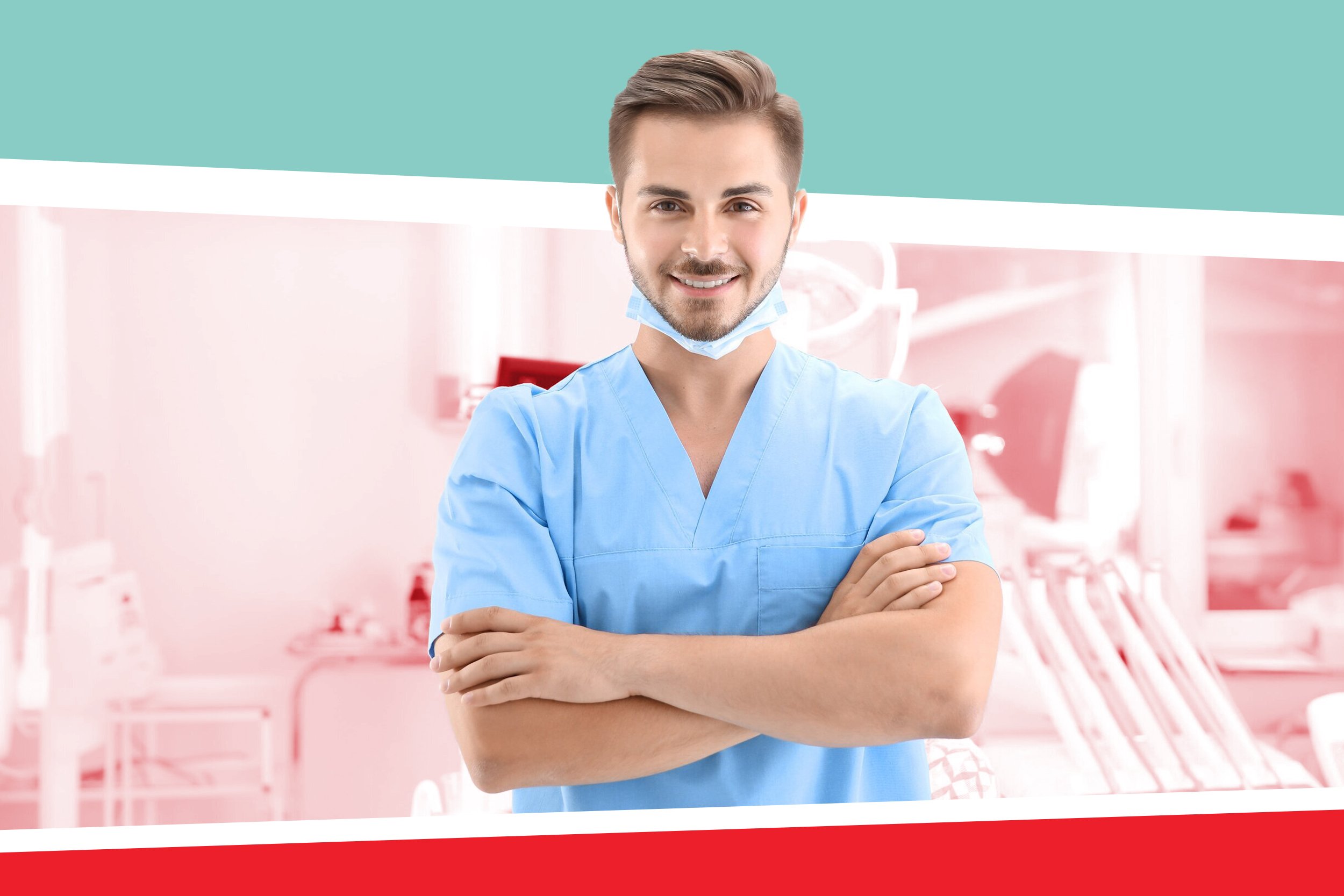This is a professional, colored photograph of a young Caucasian man, likely in his early twenties, who appears to be a medical professional. He is standing centrally in the frame, dressed in light blue scrubs. His arms are confidently crossed over his chest. He has a surgical mask tucked under his chin, revealing his light stubble beard and mustache, and his brownish-blonde hair is neatly parted and combed to the side. His brown eyes are visible, adding to his approachable demeanor. 

The background is an out-of-focus hospital room, featuring elements like an IV pole, a walker, and a hospital bed, all under a pinkish tint, contributing to the medical setting ambiance. Additionally, there are distinct color bands in the image: a blue rectangle at the top edge, with white and green stripes near the man's head, and a red stripe along the bottom of the picture. This likely indicates that the photograph may be intended for promotional use, such as a brochure or a web page, although it contains no text or additional information.